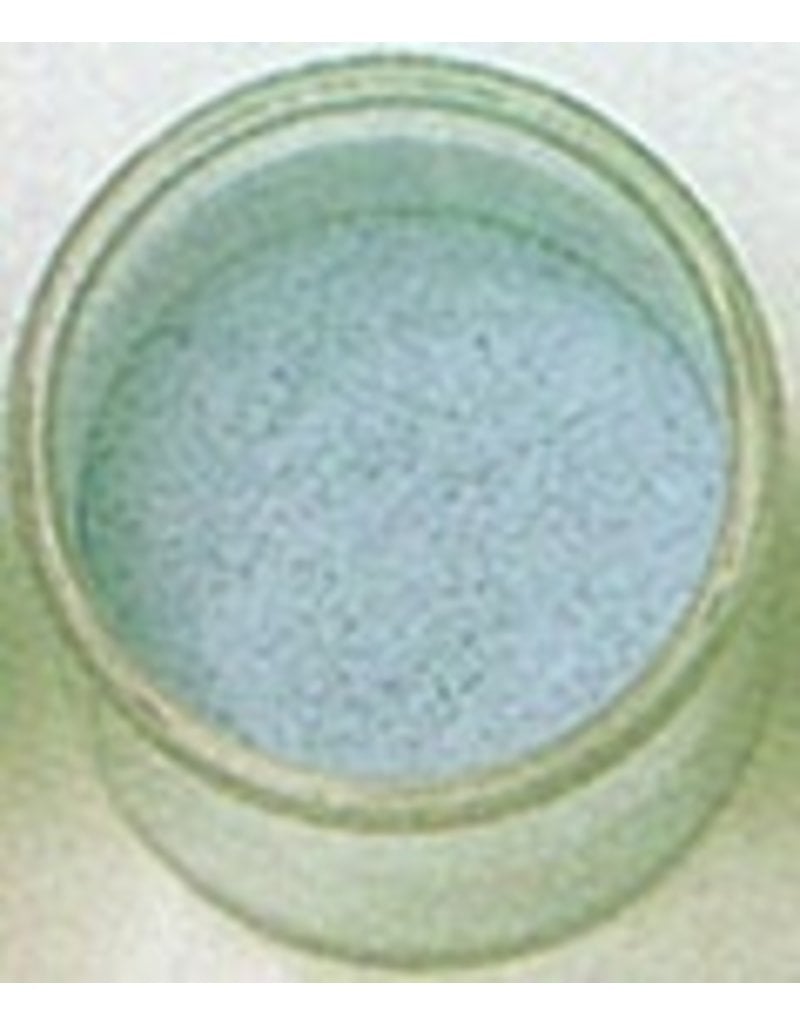The image depicts a circular container resembling a white, faded jar or petri dish, situated on a grainy, off-white surface that transitions to a shadowed, yellowy beige towards the bottom. The entire image has a grainy texture, giving it an unclear and slightly distorted appearance. The interior of the container holds a granular material that is whitish-gray, possibly sugar, rice, or flour, and there is a faint bluish tint visible within. The surrounding background is uniformly grainy with a subtle shift in lighting, brighter at the top and more shadowed below. There are no identifying texts or other objects present in the image, leaving the exact nature of the scene open to interpretation—whether it is a painting or an actual container placed on a surface remains unclear.